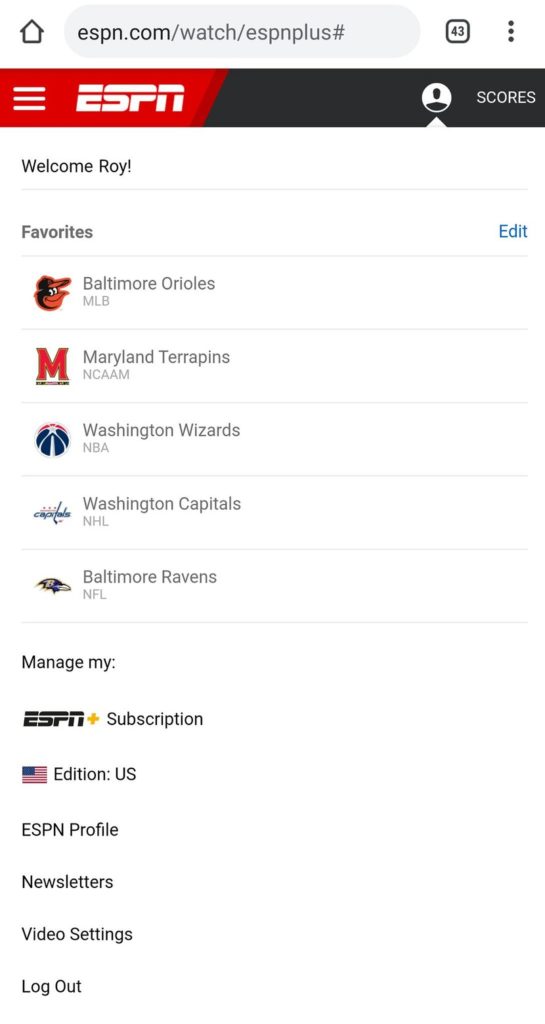The image features a clean white background with a variety of elements displayed prominently. At the top of the image is a house icon followed by a blue search box. Inside the search box, there is text that reads "ESPN.com/watch/ESPNplus#" accompanied by a small black square containing the number "43" and three dots.

To the right of the search box, a red and black box is visible. This box features three white lines and the ESPN logo. Near the edge of the black section of the box is a small white circle with an icon depicting a person's head and shoulders. To the right of this, the word "Scores" is displayed along with an upward-pointing arrow.

Below this, on the white background, the text "Welcome Roy" is visible. To the right side are the options "Favorites" and "Edit." Beneath these options is a list of sports teams and entities: Baltimore Orioles (MLB), Maryland Terrapins, Washington Wizards, Washington Capitals, and Baltimore Ravens. Below this list, there is an option that reads "Manage my ESPN Plus subscription."

At the bottom, the text "Edition: US" is accompanied by an American flag icon. Further options include "ESPN Profile," "Newsletters," "Video Settings," and "Logout."